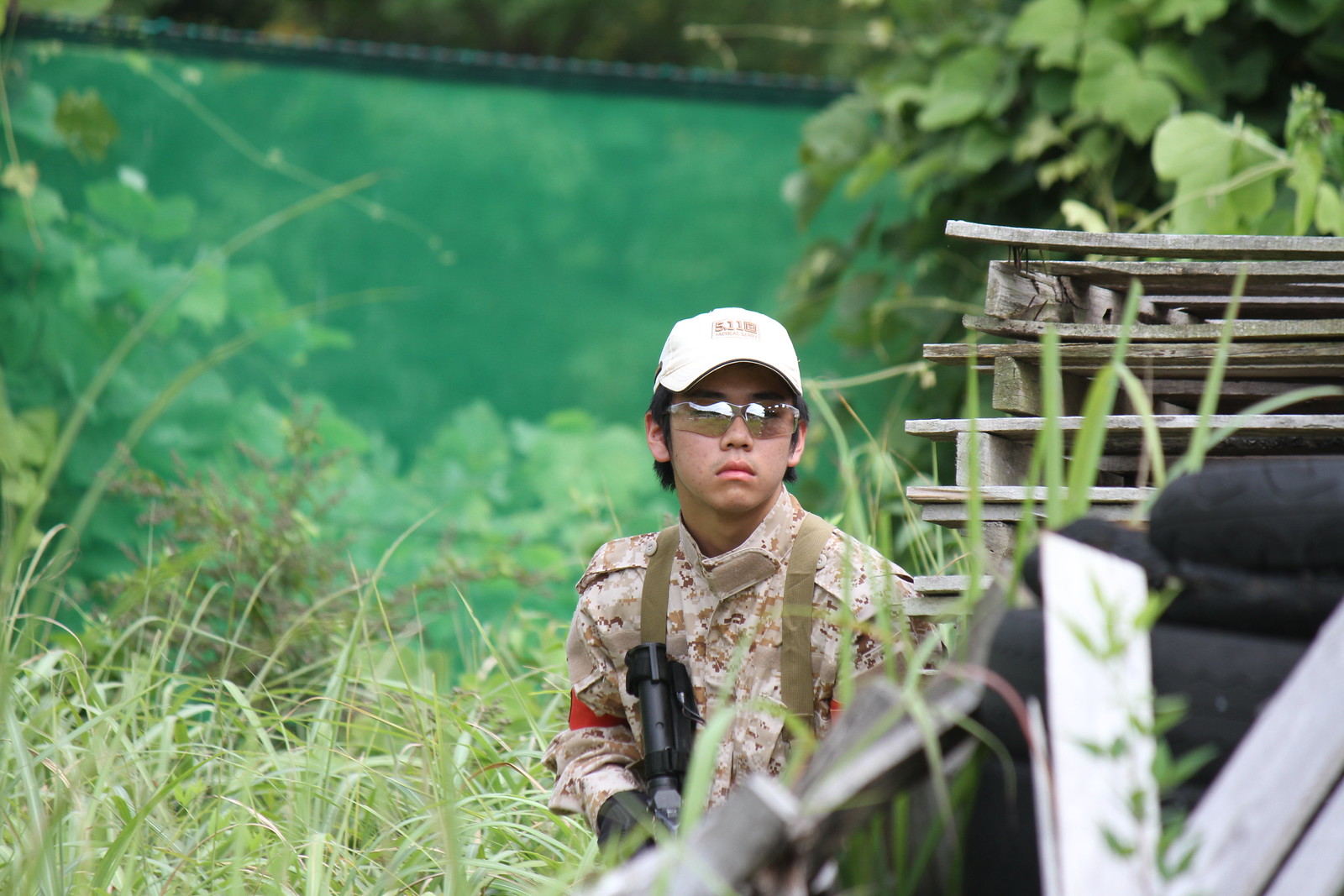A young Asian individual stands in tall green grass wearing a sand-colored camouflage jacket with light brown patches and a white hat adorned with brown numbers. He has medium-length black hair and is sporting clear protective glasses. In his right hand, he holds a black weapon, although it is unclear if it is a machine gun or a paintball gun. The background features a painted depiction of dark green plants and trees, with additional taller green plants painted in. To the right, old wooden pallets are stacked up, with a few more pallets and possibly tires in the upper right corner. Above the pallets, there are more green leaves or weeds visible.